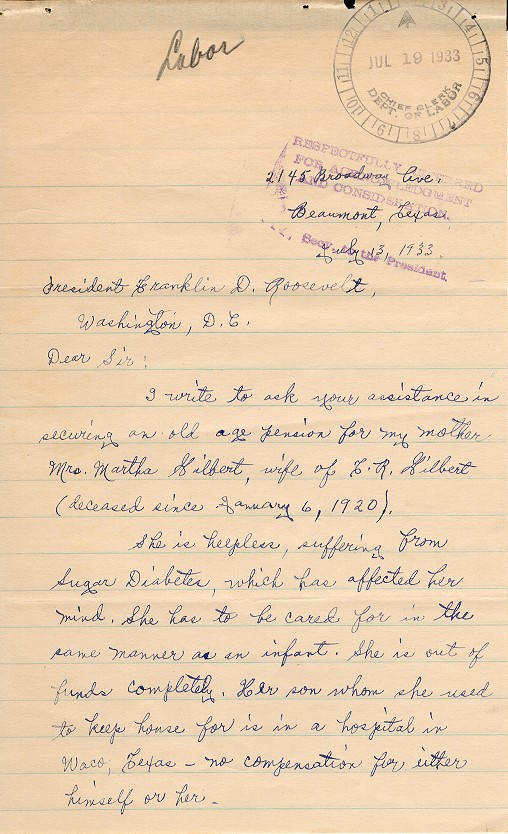The image depicts a handwritten letter dated July 19, 1933, on wide-ruled, thin-lined paper. At the top of the page, written in pencil, is the word "Labor," and on the top right corner, there is a stamp indicating "Chief Clerk at the Department of Labor." The letter is addressed to President Franklin D. Roosevelt in Washington, D.C. The text begins with "Dear Sir," and goes on to request assistance for securing an old age pension for Mrs. Martha Gilbert, who is the widow of L.R. Gilbert (deceased January 6, 1920). The writer details that Martha Gilbert is helpless and suffering from diabetes, which has affected her mentally, rendering her care similar to that of an infant. The letter further states that she is completely out of funds and her son, whom she lived with, is currently hospitalized in Waco, Texas, without receiving any compensation for his or her care.